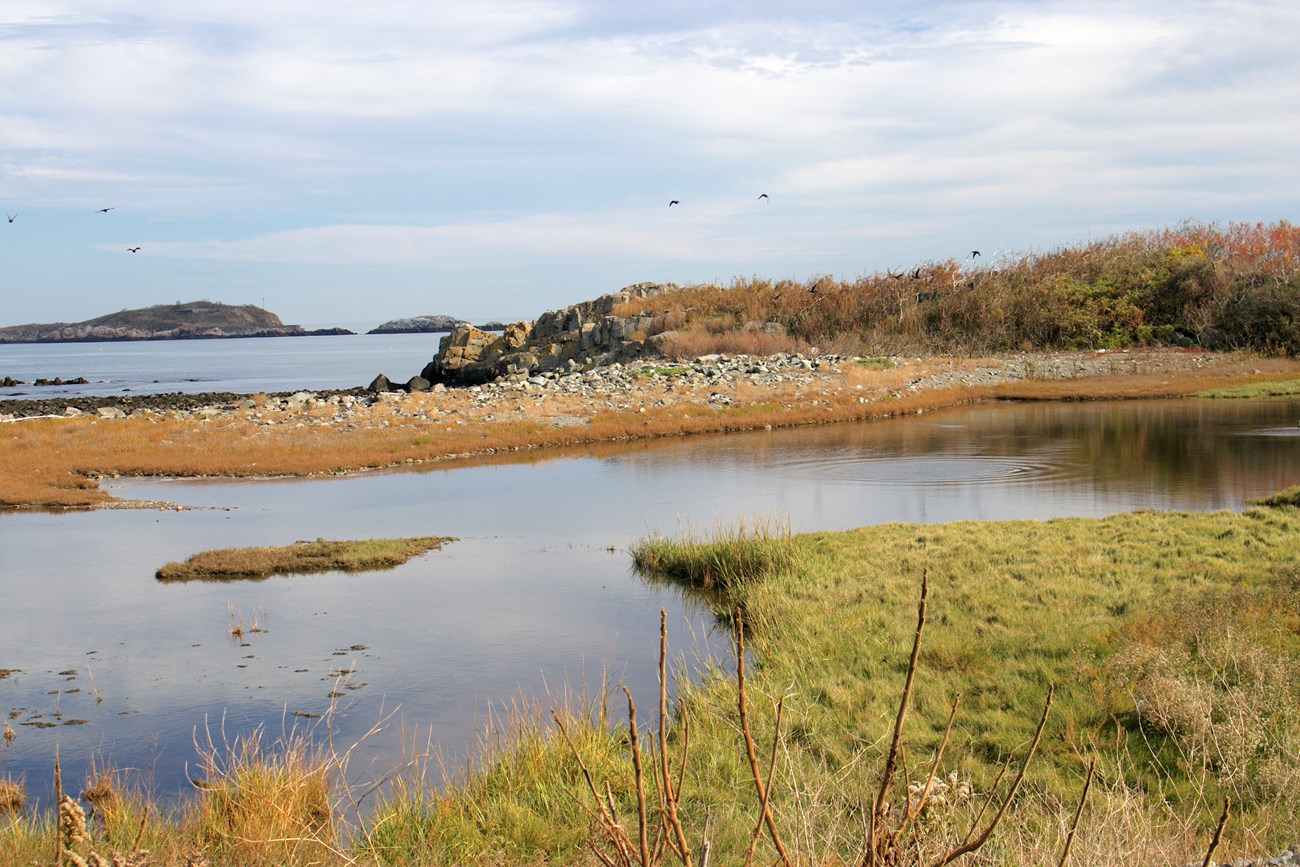In this horizontally elongated, rectangular photograph with a vintage hue, we see a serene wetland scene under a clear blue sky adorned with fluffy white clouds. The image's lower right corner reveals a grassy patch of land, transitioning into a still body of water reminiscent of a tranquil pond or small lake. From the right edge, a rocky, brown strip of land extends into the scene, juxtaposed against another expanse of water reflecting the blue sky. Along the horizon on the upper left side, hilly terrains of rocks and sparse grass rise gently. Above this grassy expanse, three black birds hover gracefully in the sky. Upon closer inspection, additional black birds can be discerned, perched among the branches and bushes dotting the land, adding a touch of life and movement to the tranquil landscape.